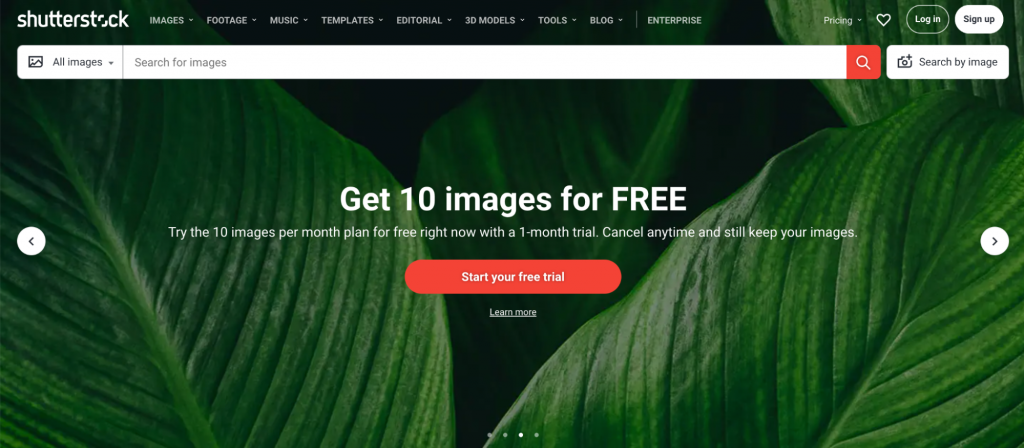The image depicts a webpage from the Shutterstock website. In the top left corner, the word "Shutterstock" is prominently displayed in white letters. Adjacent to the logo, there are several drop-down tab options including "Images," "Footage," "Music," "Templates," "Editorial," "3D Models," "Tools," "Blog," and an "Enterprise" section.

On the right side of the header, there are additional options: "Pricing," a heart icon, and a prompt to "Login or Sign Up." Below the header, a large search bar is situated. To the left of the bar, the text "All Images" is displayed, followed by the placeholder text "Search for Images." Inside the search bar, a white magnifying glass icon is set within a reddish-orange square. Adjacent to the search bar, there is a button labeled "Search by Image," accompanied by a small camera icon.

The background of the webpage features an image of lush, green leaves, evoking a serene forest setting. Across the center of this background, bold white text offers "Get 10 images for free." Below this offer, more detailed text invites users to "Try the 10 images per month plan for free right now with a one-month trial. Cancel any time and still keep your images."

At the bottom of the offer, there is a red oval button with white text reading "Start your free trial," and a smaller text link beneath it that says "Learn more." On either side of the main image, circular arrow icons allow users to navigate through the content. Additionally, four dots at the bottom of the image indicate that there are four different pages available to explore.